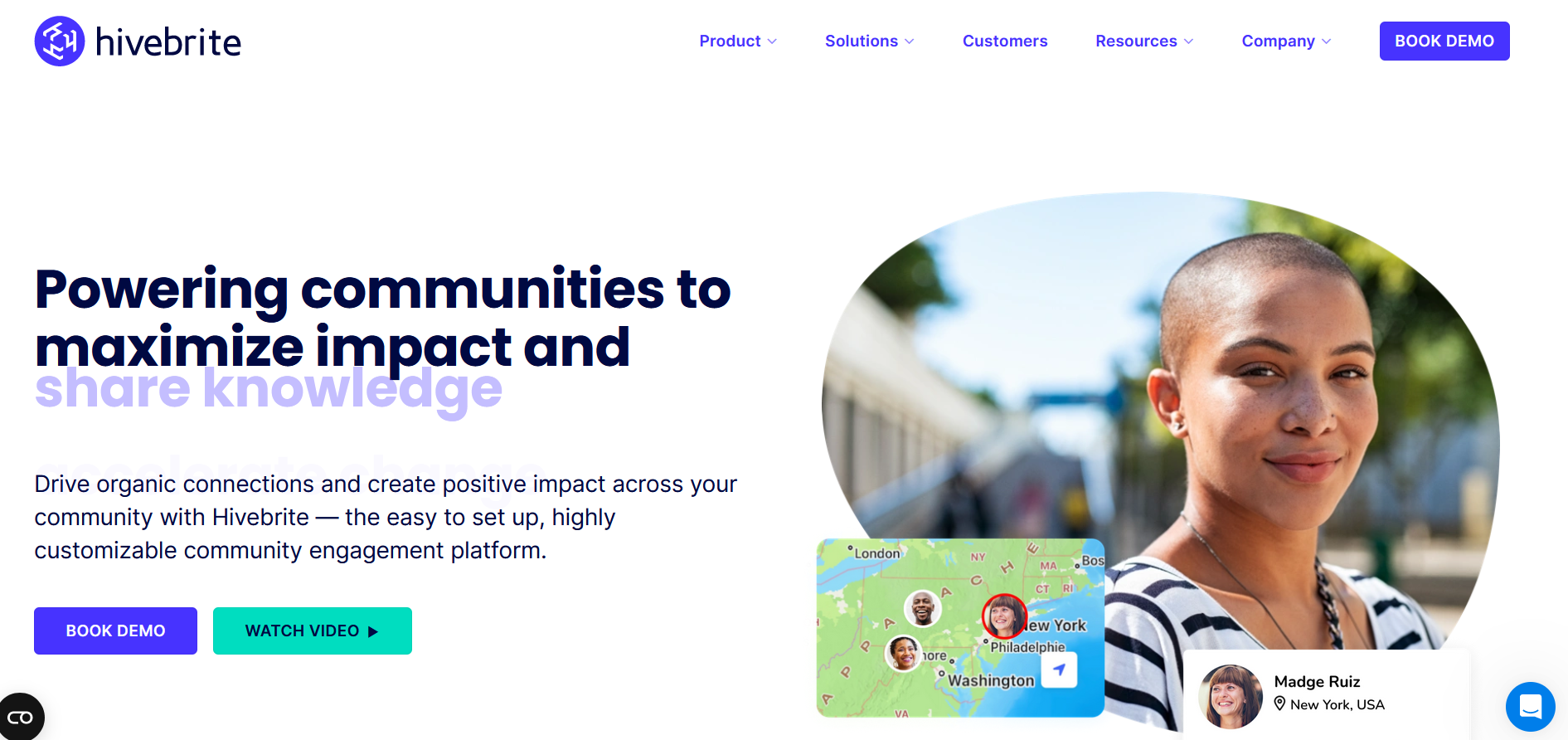This image showcases a vibrant, high-brightness website layout. The right side prominently features the website's logo alongside an icon adjacent to the site's name. At the top, a navigation bar includes tabs labeled "Product," "Solutions," "Customers," "Resources," "Company," and a bold "Book Demo" button. The tabs "Product," "Solutions," "Resources," and "Company" each have downward-pointing arrows, suggesting the presence of dropdown menus with additional options.

Below the navigation bar, a compelling tagline reads, "Powering communities to maximize impact and share knowledge." Beneath this, a detailed description states, "Drive organic connections, create positive impact across your community with a high-bright, easy-to-set-up, highly customizable community engagement platform." 

Further down, the page displays two action buttons: a dark blue "Book Demo" button and a greenish-blue "Watch Video" button. To the right of these buttons, there is a round image of a smiling bald-headed woman. At the bottom of the page, a map is visible, marked with three circular profile pictures of different individuals scattered across the map.